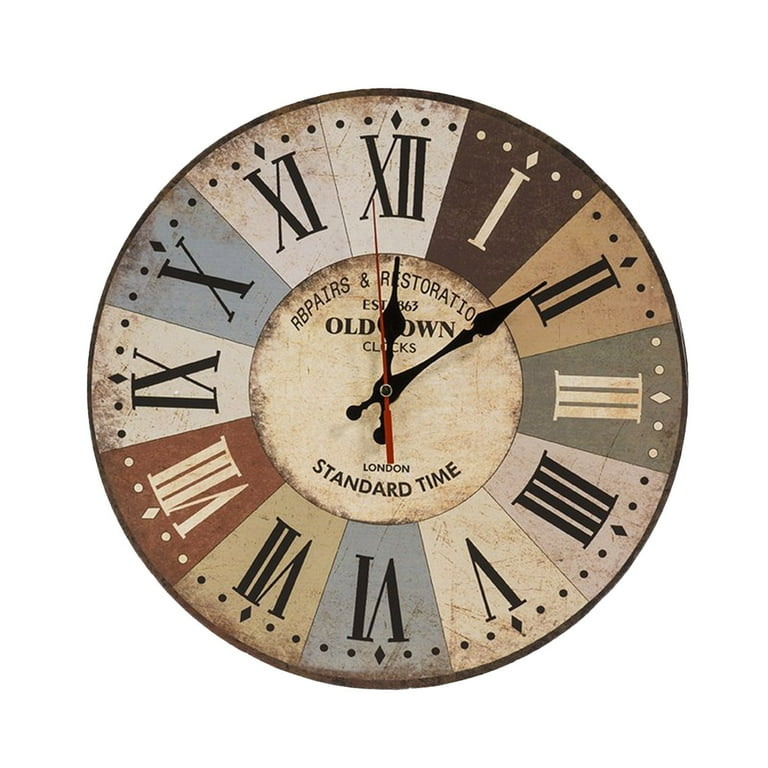This photograph captures a close-up view of a weathered and detailed round clock, with visible signs of aging, such as dirt and rust, particularly around the edges. The clock exhibits Roman numerals from I to XII on pieces shaped like trapezoids, each shaded differently: dark brown, light brown, gray, green, beige, blue, olive, and burnt orange. The hour hand points to XII while the minute hand points to II, accompanied by a red second hand. Surrounding the numerals are black and white decorations of diamonds and circles. The center of the clock features the text "Repairs and Restoration, Established 1863, Old Town Clocks," though some letters are obscured by the hour hand, followed by "London" and "Standard Time" in bent black text. The clock face's rust and weathering, particularly the brown discoloration, add to its antique charm, and a dotted border encircles the entire piece.